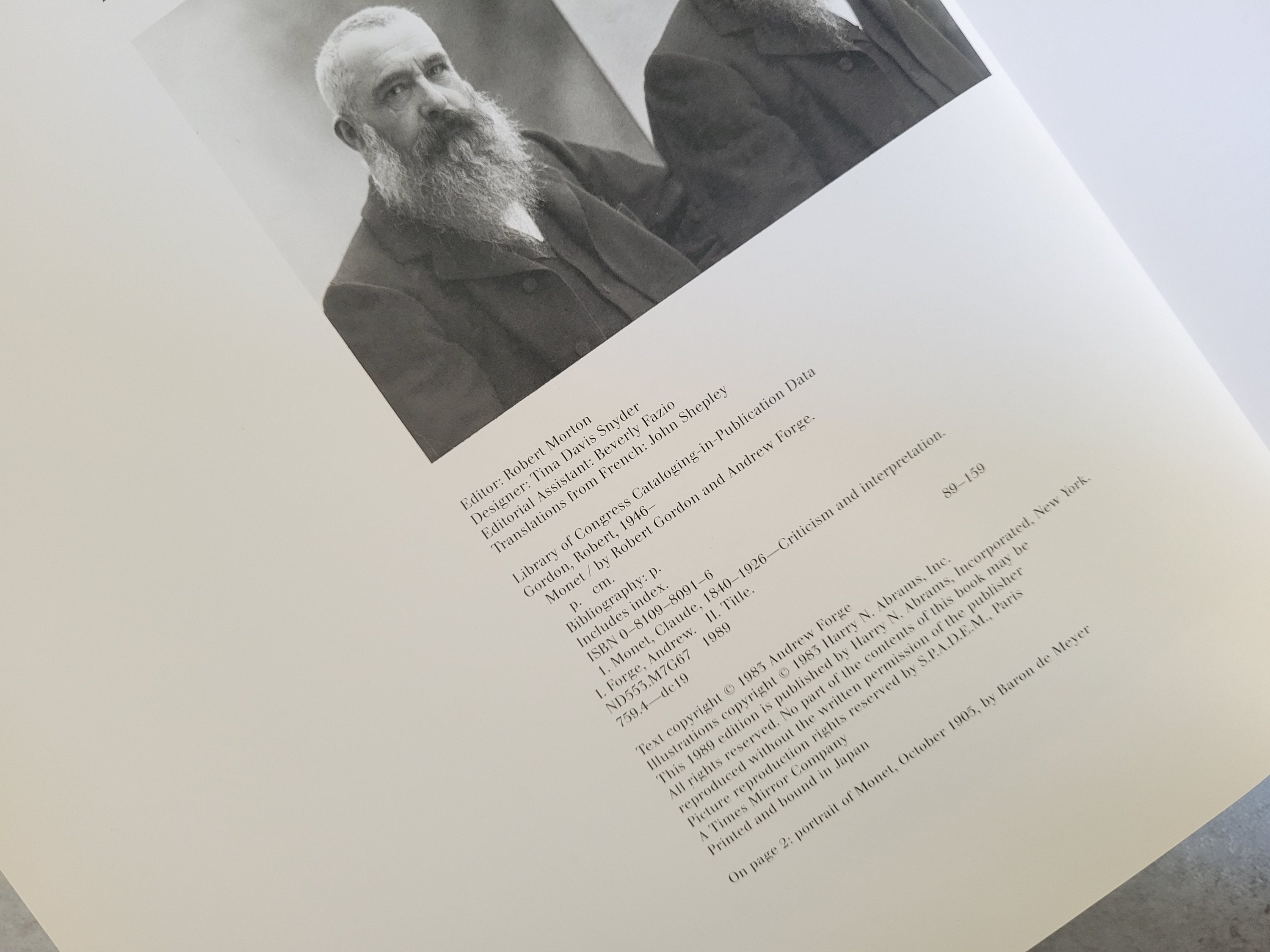A photograph of the copyright page from a book is shown, angled at about 45 degrees, revealing detailed publishing information and a sepia-toned portrait titled "Portrait of Monet, October 1905 by Baron de Meyer." The central figure, Claude Monet, is depicted with his characteristic long gray beard, dark mustache, dark eyebrows, short white hair, and is wearing a suit with a vest. The image captures Monet looking directly at the viewer. The text on the page includes editorial credits: Editor, Robert Morton; Designer, Tina Davis Snyder; Editorial Assistant, Beverly Fazio; with translations from French by John Shepley. The book's Library of Congress details list, Monet by Robert Gordon and Andrew Forge (ISBN 0810980916). The copyright mentions 1983 for both text by Andrew Forge and illustrations by Harry N. Abrams, Inc., with this 1989 edition published by Harry N. Abrams, Inc. in New York. Permissions for picture reproduction are reserved by S.P.A.D.E.M., Paris. The page itself is tan, adding to the vintage feel of the document.